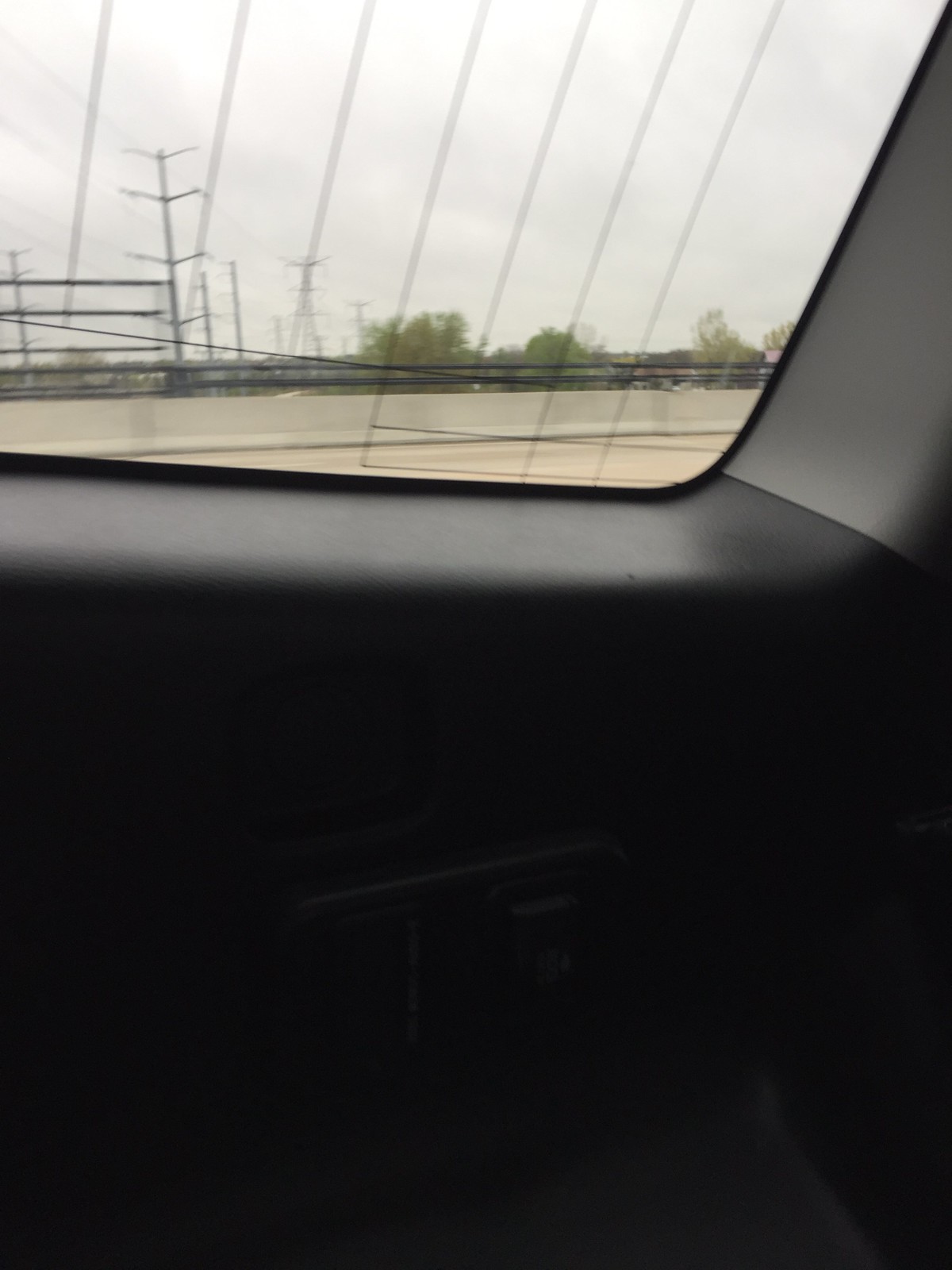This color photograph was taken from the back seat of a car, looking out the rear side window. The main feature of the interior is a dark section at the bottom, likely the back seat, with a visible handle situated in the center-bottom region. The window itself is marked by thin black vertical and horizontal lines, suggesting a defrost grid. Outside, the scene is dominated by a gray, overcast sky, hinting at imminent rain. 

In the distance, on the right side of the image, there are green trees with a sprinkling of brown among the leaves. To the left, a series of black telephone or power poles with accompanying wires can be seen, gradually diminishing in size as they stretch into the background. Additionally, there's a cement retaining wall, likely part of an overpass, visible in the middle distance, adding to the utilitarian landscape. The image captures a somber, cloudy day, with no people, animals, or signage in view.